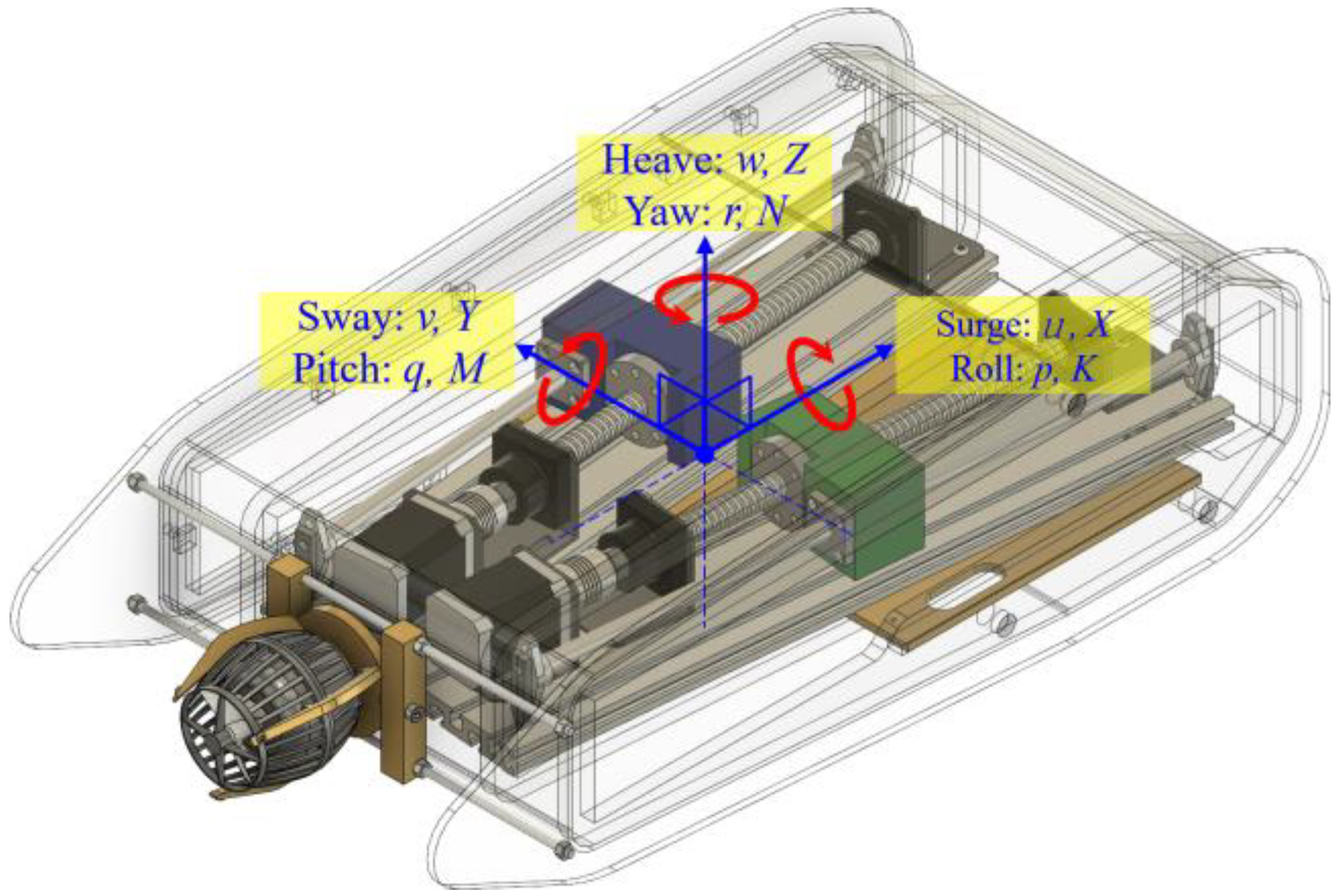The image depicts a detailed, transparent schematic of a machine, resembling a briefcase shape with rounded edges, oriented diagonally from the bottom left to the top right corner. The outline allows a view of its intricate inner components. Central to the drawing are two elongated screws, one blue and one green, positioned vertically and flanked by horizontal metal posts. These screws are capped with black bolts at their tops and continue through various mechanical parts within the machine.

Situated at the bottom left of the image is a fan-like propeller, possibly metallic, attached to a set of interconnected wooden and metal posts. Directly above these screws, explanatory labels are indicated by blue arrows and accompanied by red-circled annotations. These labels are enclosed in opaque yellow boxes with blue text and denote various mechanical axes and movements: 

- The middle box, pointed to by an arrow from the center blue dot, reads "sway: V, Y" and "pitch: Q, M."
- A second box is positioned higher, with an arrow pointing upward from the central dot, and reads "heave: W, Z" and "yaw: R, N."
- A third box, reached by another diagonal arrow pointing up and to the right, is labeled "surge: U, X" and "roll: P, K."

Additionally, multiple dashed lines extend from this central blue dot: one downward, one diagonally down to the left, and another diagonally down to the right. A bowtie shape is depicted, extending upwards from about one-third of the length of the middle arrow.

The outer casing of the mechanism is transparent, further showcasing internal features such as springs, knobs, and miniature barrels. These components, alongside the labeled axes, suggest a complex mechanism, the function of which is indicated through its detailed anatomical breakdown.